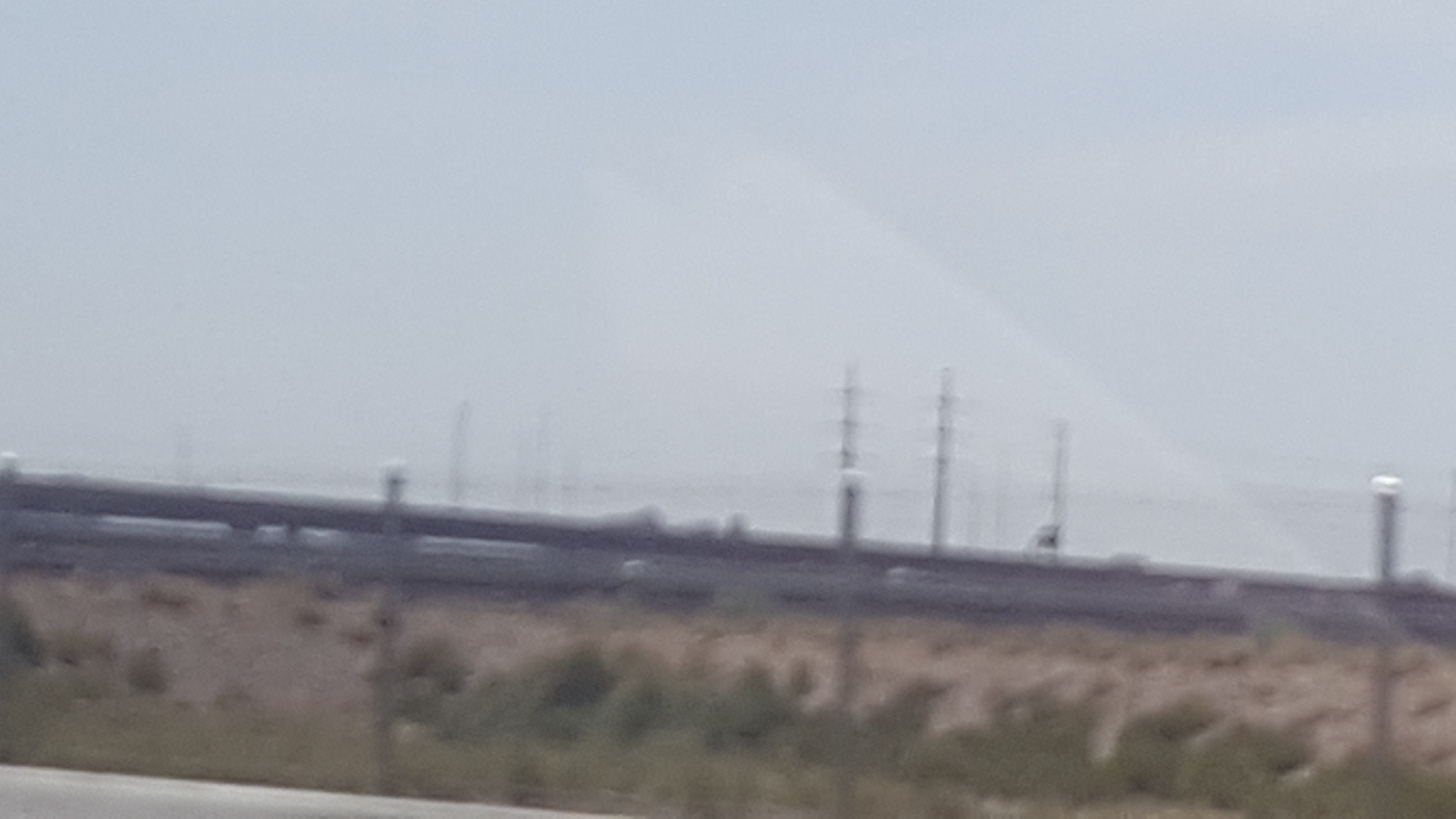This daytime photograph, though slightly blurry and grainy, captures a snapshot of a small roadside scene. In the foreground, a portion of a road is visible, bordered by patches of green bushes, uneven grass of varying heights, and some exposed dirt. Further back, the image hints at a guard rail, though it is out of focus. Silver poles, topped with rounded white objects, possibly streetlights, are also faintly discernible. Power lines stretch across the far background, adding to the urban aspect of this setting. Additionally, there is a glare from the light that partially obscures the view, and a few cars are faintly visible, hinting at distant traffic.